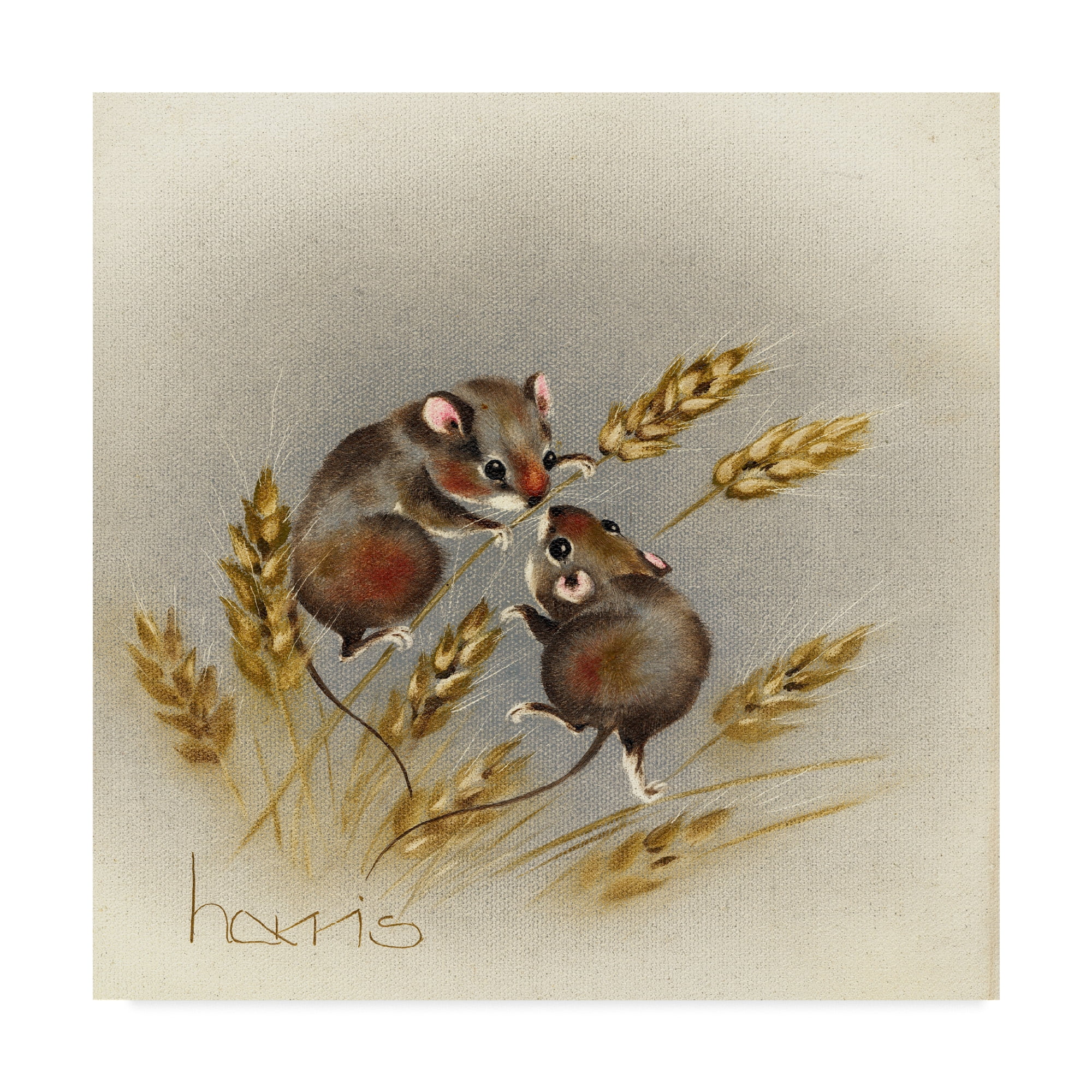This artwork, signed by Harris, is a detailed painting or print on a square canvas showcasing two brown, fluffy field mice with pink ears, beady black eyes, and white undercoats, paws, mouths, and areas around their eyes. They also have hints of red coloring on their cheeks, noses, and other parts of their bodies. One mouse, characterized by a particularly red nose and cheeks, clings to a golden wheat stalk, which features delicate white feathering and pine cone-like ends. The other mouse appears to be mid-jump, reaching towards the first mouse as if trying to touch noses, but just out of reach. Both have short little tails. The background of the canvas is textured with leaves and features a gradient burst from light gray in the center to whitish hues at the edges, giving the image a soft, circular framing. The artist's signature, Harris, is stylized and located at the bottom right, adding a finishing touch to the charming scene.